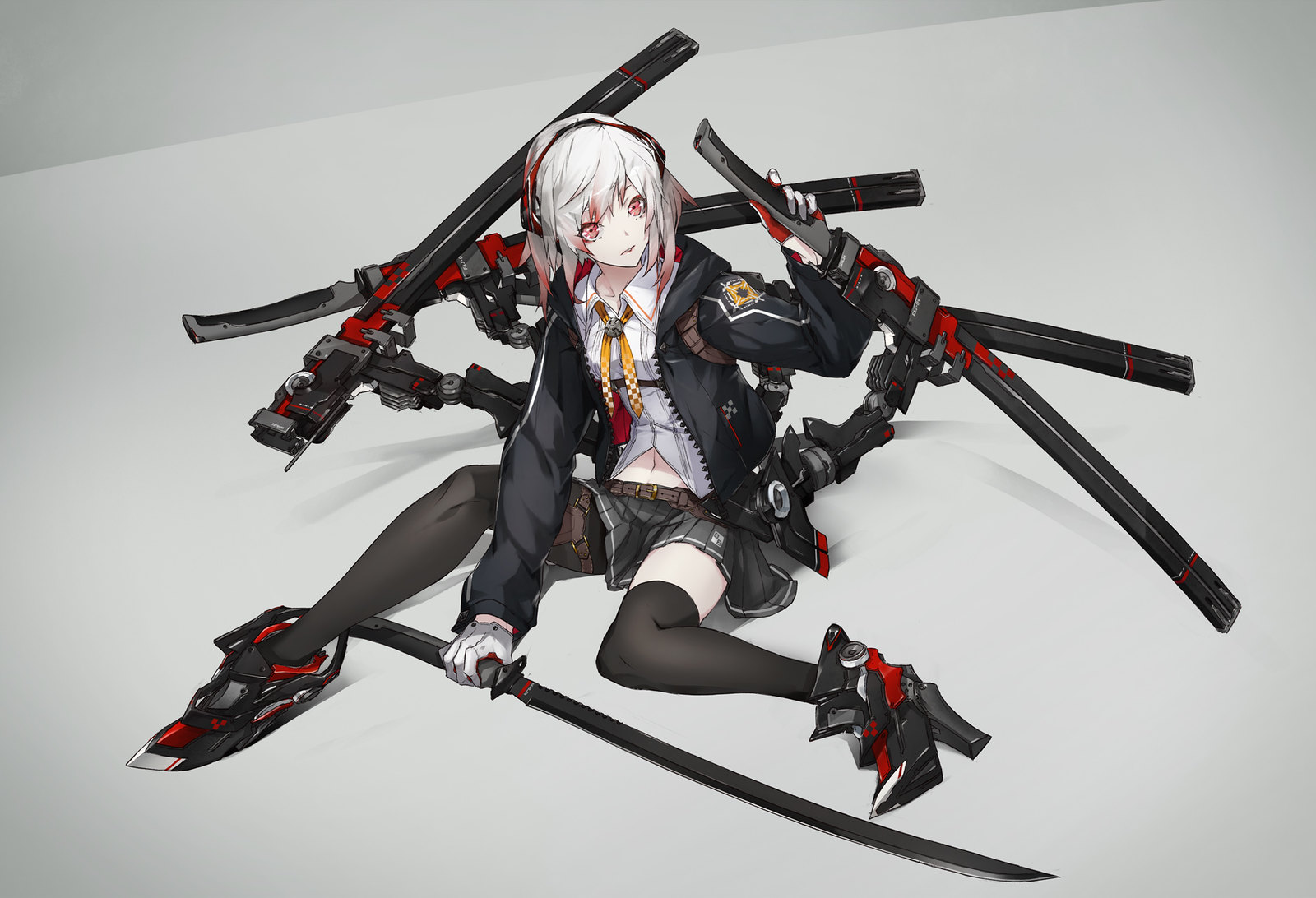In the center of a mostly gray background, an anime-style teenage girl sits, embodying a futuristic warrior aesthetic. She has striking white hair with red tips and piercing red eyes. Dressed in a short, pleated gray skirt and a button-up shirt with a collar, she exudes a blend of schoolgirl innocence and combat readiness. Over her outfit, she wears a black hoodie adorned with various weapons and swords, hinting at her warrior capabilities. Her futuristic ensemble includes black thigh-high stockings, accessorized with a garter, and distinctive high-heeled shoes that feature metal armor and red accents, resembling a meld of dress shoes and boots. Additionally, she possesses multiple arms, each carrying a sheathed sword, and there are extra mechanical limbs and blades emanating from her back, enhancing her combat-ready appearance on the monochromatic stage she occupies.